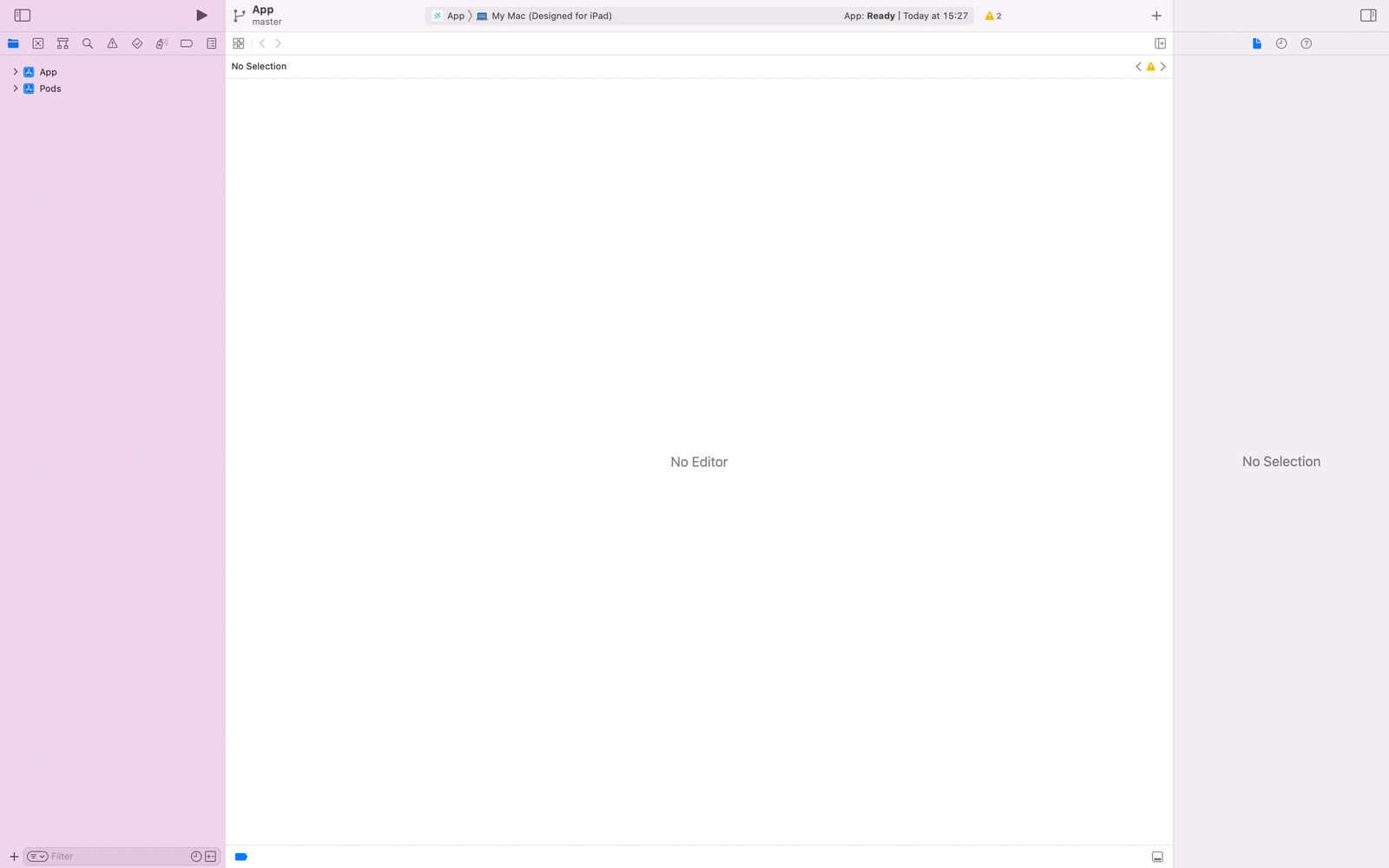A screenshot of a software development application is depicted, showcasing its user interface. The application features a purple-hued sidebar located on the left-hand side, adorned with various icons including a play button at the top right, a folder icon, a search icon, and several other indistinguishable icons. Below these icons, expandable menus labeled as "apps" and "pods" are present. The central panel, with a white background, displays text that reads: "app master, app, expanded to my Mac, designed for iPad, app ready today 15:27," accompanied by the phrases "no selection" and "no editor here." The right-hand panel, shaded in gray, similarly notes "no selection," completing the interface layout presented in the screenshot.